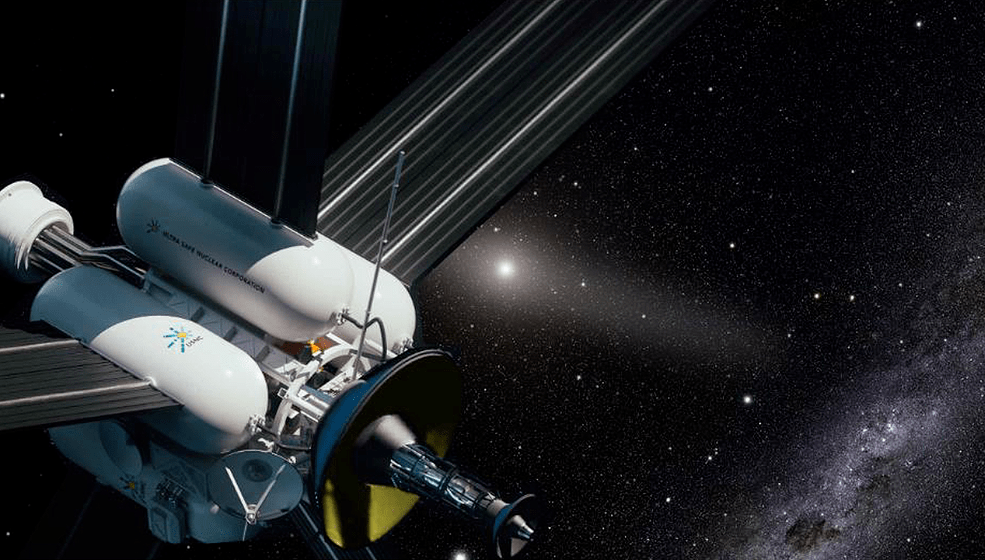This vibrant, horizontally rectangular digital artwork captures a detailed scene set in the vastness of outer space. The background features a striking contrast of deep black space, densely populated with twinkling stars of varying sizes, including a prominent, luminous star at the center that emanates light throughout the image. 

The left side of the piece is dominated by an artistic depiction of a satellite. This complex structure comprises an intricate arrangement of white tubes forming a round assembly. Additionally, there are three noticeable solar sails extending to the top, left, and right, while an antenna and a yellowish satellite dish are positioned centrally within the satellite, complete with an extender protruding outward.

In the lower right-hand corner, there's an intricate cluster of stars, creating the impression of a separate galaxy, some of which are enveloped in smoke-like white clouds with hints of brown, enhancing the depth of the cosmic vista. The satellite's components, such as rectangular fans or blades with distinctive black and white striped patterns, cast subtle shadows, hinting at the intricate detailing of the artist's work.

The artist masterfully integrates these elements, providing a captivating visual representation of a satellite navigating through the celestial expanse, capturing both the majesty and mystery of space exploration.